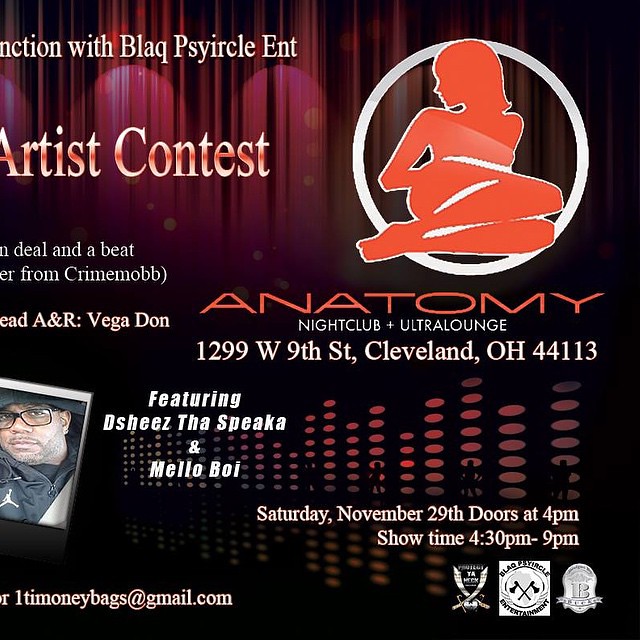The poster is an advertisement for the Anatomy Nightclub and Ultra Lounge in Cleveland, Ohio, located at 1299 W 9th Street, Cleveland, OH 44113. The backdrop features a deep crimson curtain. Dominating the upper right section is the club's logo, a white circle encasing the orange silhouette of a reclining woman. Below the logo, the club's name, "Anatomy," is prominently displayed in modern orange lettering, accompanied by "Nightclub Ultra Lounge" in white text.

The left side of the poster has the text and a small image of an African-American gentleman, sporting glasses and an Air Jordan outfit, identified as "Dashiz the Speaker." The poster also mentions another performer, "Mellow Boy." Additional details, such as the date, "Saturday, November 29th," the address, and the event time, "Doors at 4 p.m., Showtime from 4:30 p.m. to 9 p.m.," are written in white at the bottom, along with an email address for contact. The design prominently uses orange and white fonts against the rich red curtain background to create a visually striking promotional piece.